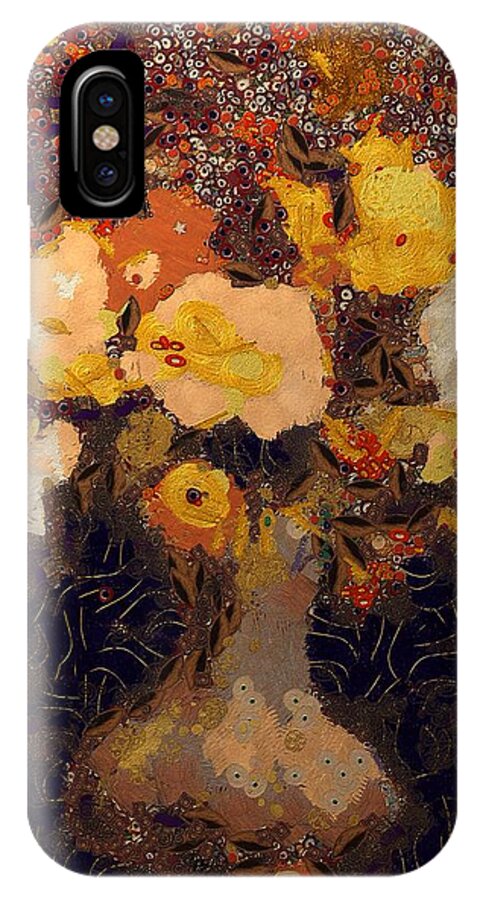This photograph showcases the back of a regular-sized smartphone, highlighting its hand-painted DIY design. The phone itself, a rectangular shape with beveled corners, is about five inches high and three inches wide and appears more illuminated on the left due to a light source. The upper left corner features a prominent black oval housing a vertically aligned set of camera lenses and a flash. The back design, possibly a mosaic or abstract representation, depicts what resembles a tree with multi-colored foliage. At the bottom, the design is dark with black interlaced patterns, transitioning upward through a tree trunk-like section. The vibrant colors include black, brown, red, orange, yellow, and beige, with large flower shapes at the base becoming smaller white and orange circles with black and yellow dots as they ascend. The overall effect is an imaginative and intricate artwork, blending various hues and shapes to create an eye-catching visual on the smartphone case.